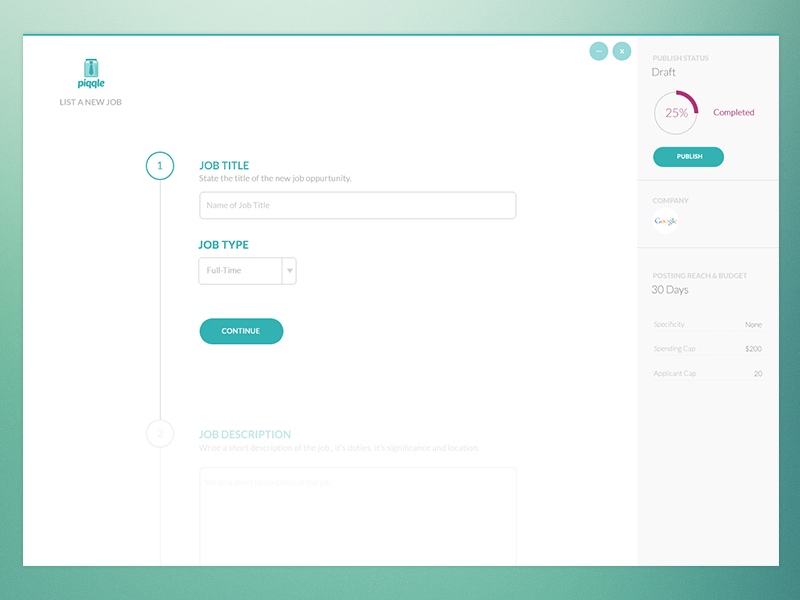The image is a horizontally oriented rectangle with a clean white background, bordered by a bold green line featuring varying shades of green. In the top left corner, there's an icon labeled "PIGGLE" in uppercase letters. Below this icon, there is gray text that reads "List a new job," followed by a circled number "1" that introduces the section titled "Job Title."

The section prompts the user to state the title of the new job opportunity and provides a blank text box labeled "Name of Job Title." Directly below, there's a section titled "Job Type" with a pull-down menu, which currently has "Full Time" selected. Adjacent to this menu is a prominent blue circle labeled "Continue."

Further down, faint text introduces section "2. Job Description," instructing the user to write a short description of the job, its duties, significance, and location, followed by another blank text box designated for this information.

On the right-hand side of the image, there is a pale gray column detailing the publication status, which indicates "Draft, 25% completed." Below this is a blue oval button labeled "Publish." Additional information in the column includes the company name "Google," hosting platform, reach, and budget specifics: 30 days, applicant policy with specificity marked as "None," a spending cap set at $200, and an applicant cap of 20.